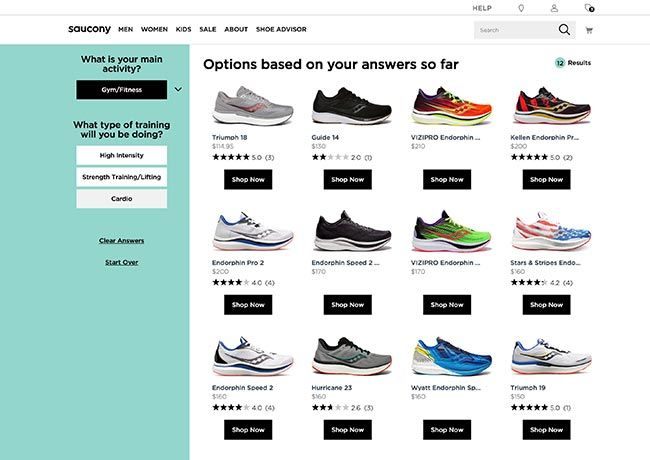The image captures a detailed layout of a webpage from the shoe-selling company Zirconi. At the top of the page, the Zirconi brand is prominently displayed, along with a navigation bar offering sections for Men, Women, Kids, Sale, About, and Shoe Advisor.

On the left side of the page, there is a distinct teal rectangle box featuring a dropdown menu with the prompt "What is your main activity?". The dropdown menu currently displays "Gym, Fitness" in a black box, indicating that users can select their primary activity. Following this, another query asks, "What type of training will you be doing?", offering options such as High Intensity, Strength Training, Lifting, or Cardio. Below these queries, there are buttons available to "Clear your answers" or "Start over."

In the central section of the webpage, there is an organized display of shoes arranged in three rows, with four pairs of shoes in each row. Each shoe entry includes an image of the shoe, the shoe's name, its price, a rating depicted by stars, and a black box labeled "Shop Now" in white print, allowing customers to make a purchase directly.